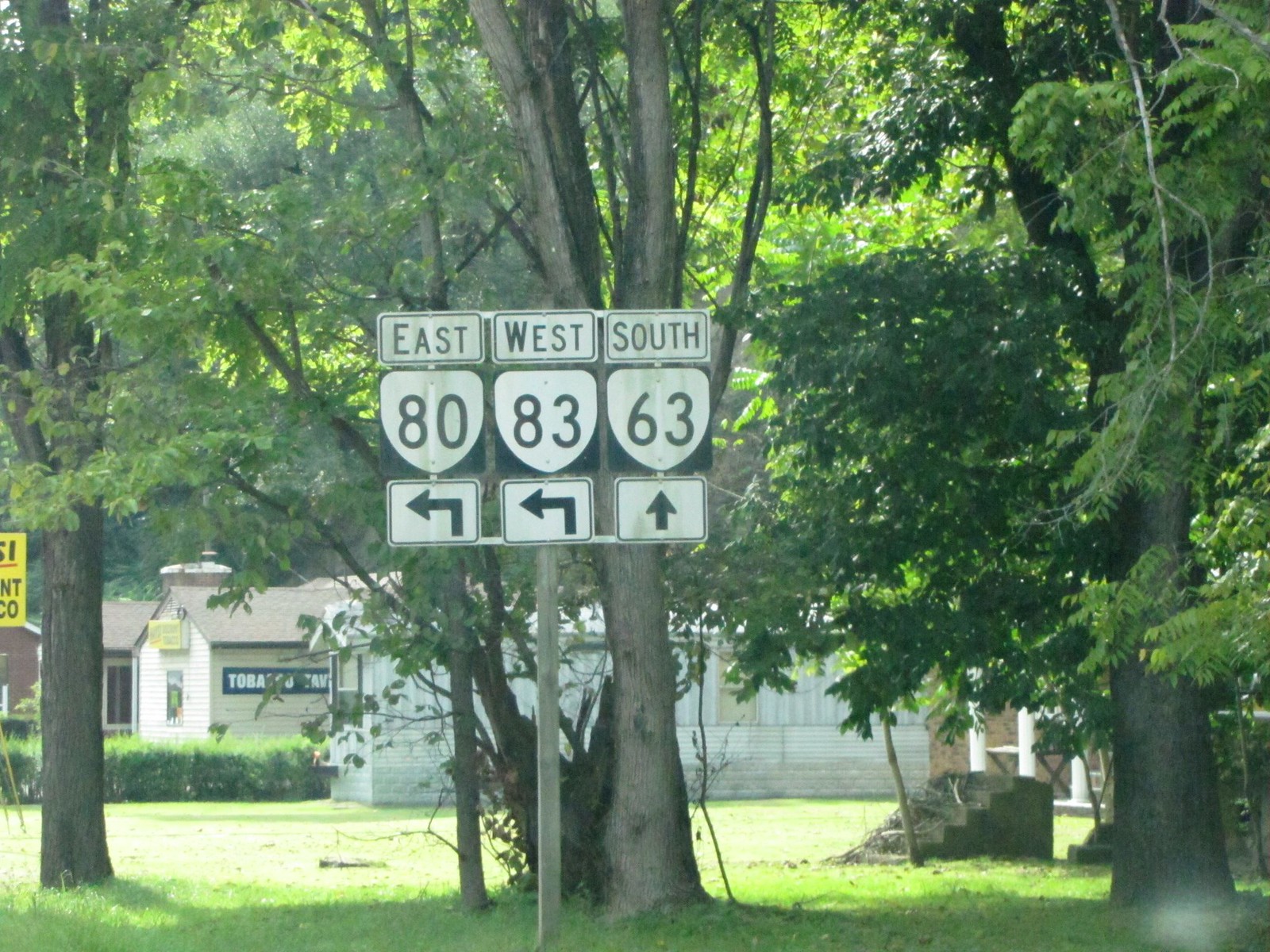In this rectangular photograph, the top and bottom sides are longer than the left and right sides, providing a wide view of a cluster of street signs set against a backdrop of a neatly trimmed green lawn. At the center of the image stands a slim, cylindrical gray metal pole anchored in the grass. This pole features a white bracket positioned at the top and the middle, supporting three distinct signs.

The leftmost sign is rectangular with a white background and a bold black border. It prominently reads "EAST" in large black letters. Directly beneath this is a square sign showcasing a white shield with the black numerals "80" inside, indicating a route number. Finally, underneath the shield, there is another rectangular sign bordered in black, featuring a left-pointing arrow to guide drivers. The layout and clear visibility of the signs imply a specific directional guidance system for travelers.